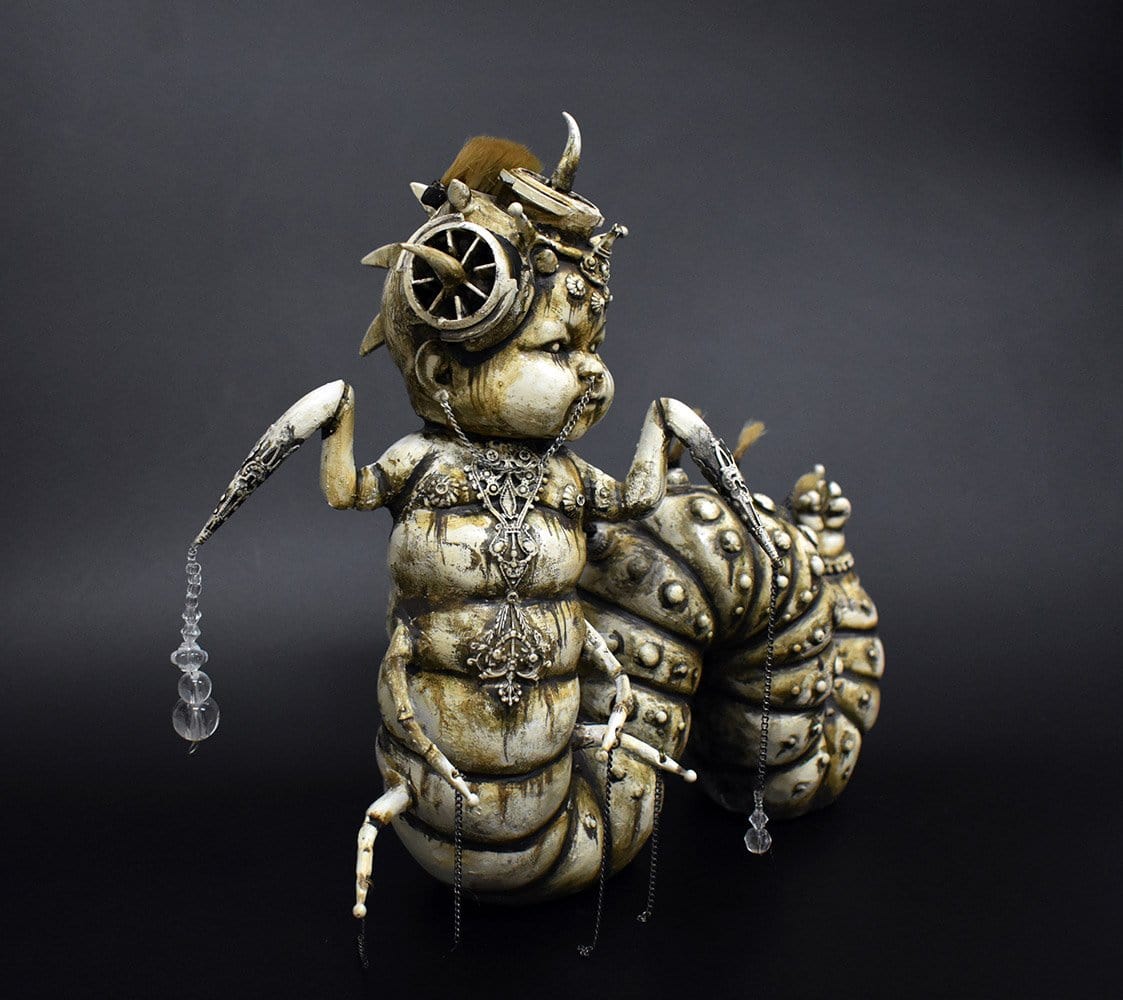This image showcases an unusual, highly detailed sculpture that features the head of an infant child attached to a segmented caterpillar-like body with pointed, bug-like legs. The sculpture is primarily in varying shades of gray and tan, showcasing significant texture with visible signs of wear and tear. 

The infant's head is adorned with a chain connecting a nose piercing to an ear piercing, and an elaborate pendant hangs down to approximately the mid-torso. Notably, there are horns arranged in a circular formation atop the head, and a small wheel or circular element is attached to the side, with hair sprouting from this area. Additionally, the head is slightly tilted to the right.

The right arm—resembling that of an insect—features a chain adorned with clear jewels, giving the impression of jewelry. Meanwhile, the left arm, similar in form, appears to be dripping with translucent resin or clear bubbles. The entire sculpture is meticulously crafted, set against a stark black background which accentuates its intricate and peculiar design.